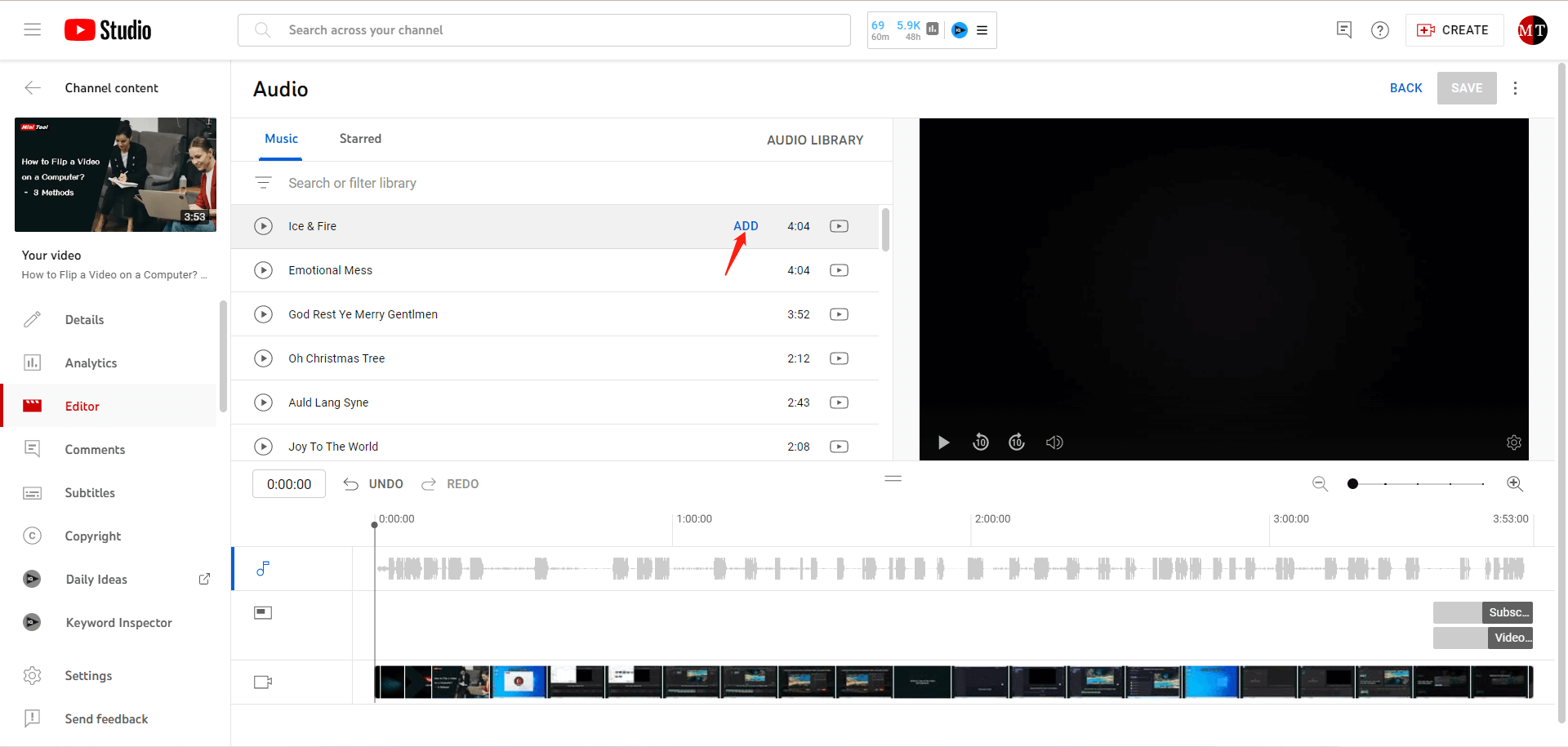The image depicts a YouTube Studio interface. Dominating the upper left side is a red box with an arrow, accompanied by the text "Studio" in bold black letters, indicating that the interface indeed belongs to YouTube Studio. At the top of the screen, there is a search bar labeled "Search across your channel," emphasizing that the platform in use is YouTube. Just beneath the search bar, a blue arrow points to a box containing blue text. 

On the upper right-hand corner, the options "Create" and "M/T" (Manage/Tools) are visible. A notable image on the left side features two businesswomen positioned at a desk or podium. Below this image, there's a heading labeled "Your Videos," followed by titles such as "How to flip a video on a computer."

Additional interface elements include sections for "Details," "Analytics," and an "Editor" highlighted in red. Navigation options like "Conferences," "Subtitles," "Copyright," "Daily Ideas," "Keyword Inspector," "Settings," and "Send Feedback" are also present.

Centrally located on the interface, the word "Audio" is displayed prominently with the subsection "Underwriting Music" highlighted in blue. A gray-highlighted box with the word "Add" inside is marked by a red arrow directing attention towards it. Below this, you'll find visual representations of song lyrics or beats—depicted as gray blocks which presumably track the rhythm.

In the upper right corner of the interface, a black box houses an interactive arrow that users can click to view a video.